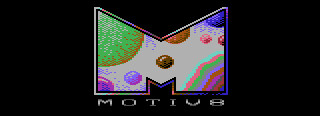The logo features a prominently designed, bold letter "M" set against a black background. The main body of the letter "M" is white, which serves as a canvas for a vibrant array of shapes in multiple colors including green, blue, purple, brown, orange, and red. These colorful shapes, resembling planets or celestial objects, are intricately positioned within the contours of the "M," adding a dynamic and cosmic feel to the design. Below the letter "M," the text "M-O-T-I-V" followed by the numeral "8" spells out "Motivate" in a cohesive and stylish manner, encapsulating the theme of inspiration and energy conveyed by the logo.